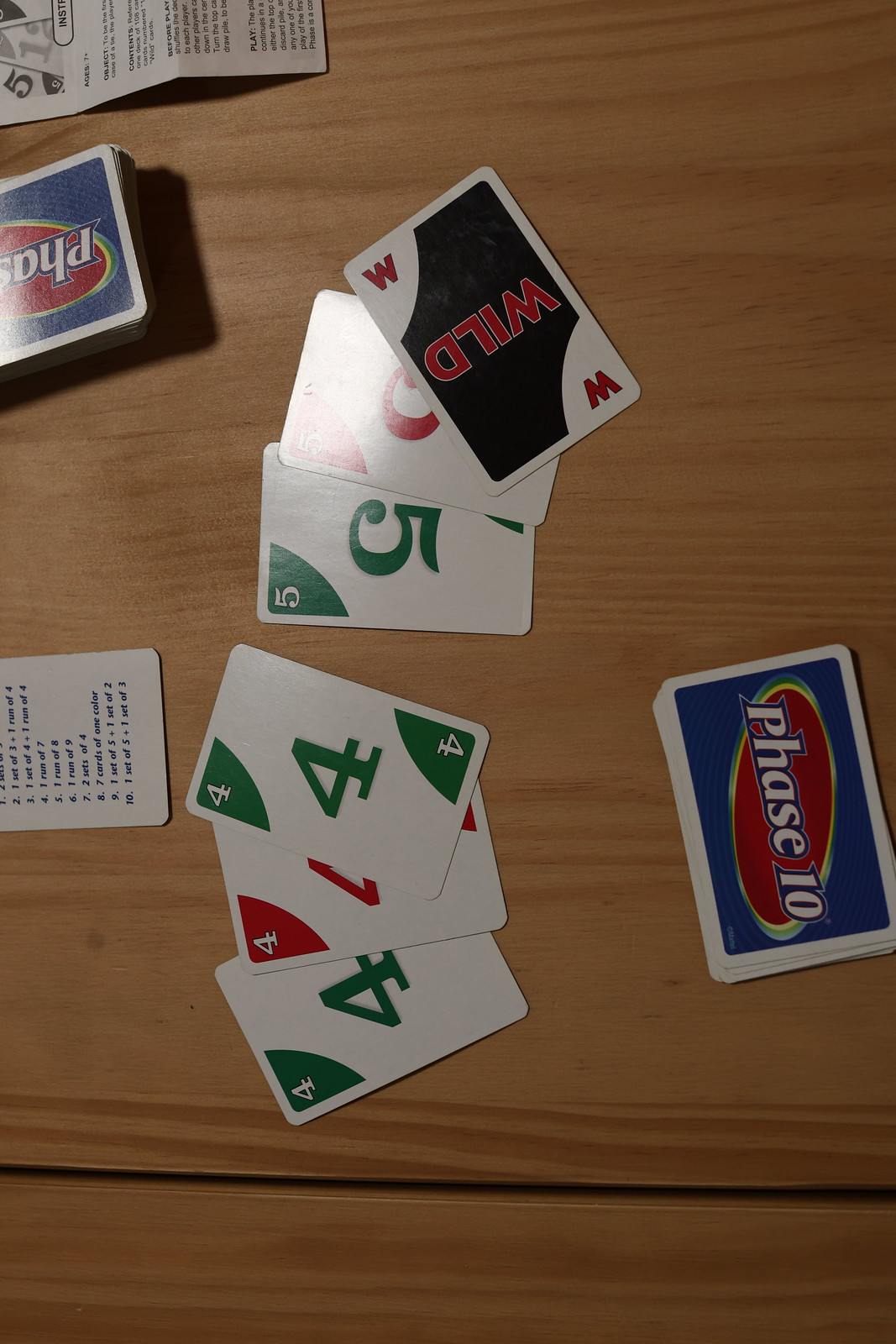An aerial shot features a blonde pine table, clearly divided into two sections with a visible separator towards the bottom horizontal line. The table hosts an array of playing cards from the game Phase 10, showcasing a colorful mix primarily dominated by red, green, and white hues. Notably, at the lower right corner, there is a stacked set of cards with the top card's back displaying the "Phase 10" logo, encased in a red oval surrounded by yellow, against a predominantly blue background framed by a white border.

Further examining the cards from top to bottom, we first encounter a "wild" card in red with a black border, marked by "WW" on each corner in red. Next, a sequence of cards follows: a red "5", a green "5", a green "4" stacked partially over a red "4" and another green "4." To the top left, another card from the Phase 10 deck is visible, lying near what appears to be a receipt positioned roughly in the middle on the left side of the table. The detailed placement and varied colors of the cards create a dynamic and engaging scene.